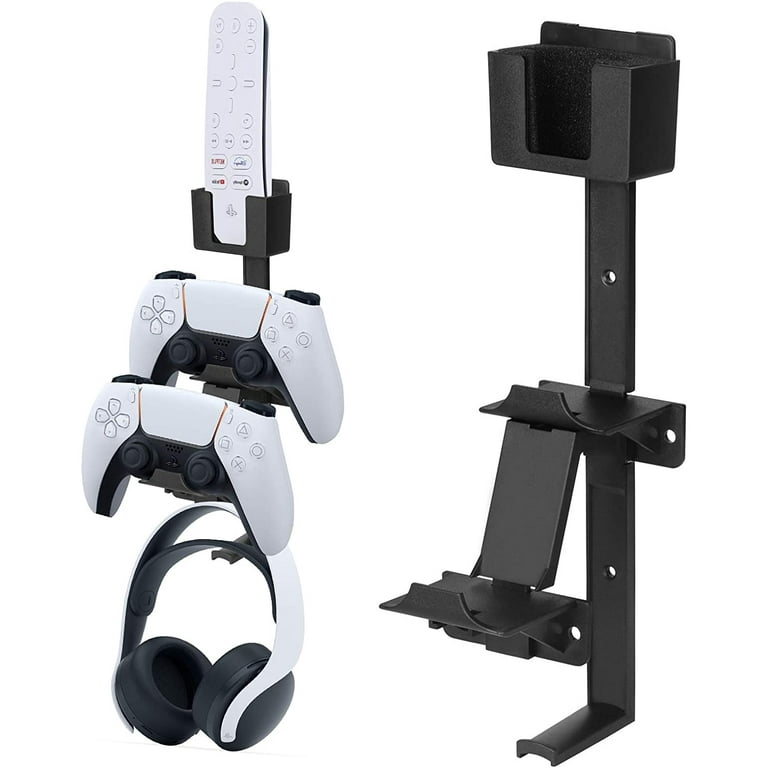This photograph showcases a sleek and functional black metal storage rack designed for avid gamers to neatly organize their gaming equipment. The rack, featured in a catalog or e-commerce listing, is built with a sturdy spine and four shelves, each serving a specific purpose. At the bottom, there's a hook for hanging PlayStation headphones. Moving up, the next two shelves are intended for PlayStation controllers, with the lower shelf slightly in front of the one above to accommodate the two controllers ergonomically. At the top, there is a small slot to vertically place a remote control. The product's design incorporates screw mounts for easy installation on a desk or wall, and features holes at the back for cable management, allowing users to charge their devices while they are mounted. The entire assembly has a clean, modern aesthetic with a black and white color scheme, with official Sony peripherals pictured to demonstrate its usage.